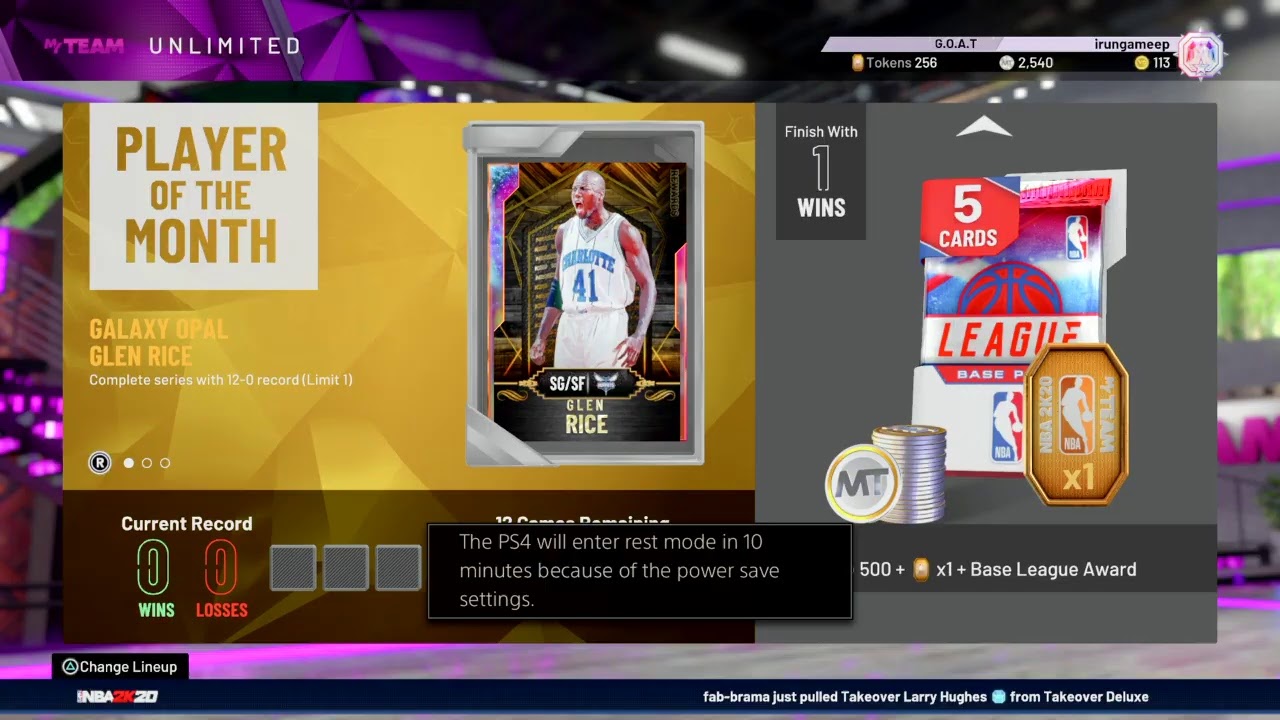This is an NBA-themed screenshot, possibly from a video game on a laptop or desktop computer. The image is significantly wider than it is tall, with a multicolored background featuring a blend of purplish-violet on the left and gray on the right. The background image, vaguely discernible as a room, is lit up with blue hues on the left side but is largely obscured by various elements. 

In the upper left corner, there is a violet logo with "MY TEAM" written on it, and next to it, in all caps white letters, "UNLIMITED". The upper right corner displays the text "G.O.A.T." followed by "iRUNGAMEEP". Below this, it indicates the user has 256 tokens, denoted as "tokens: 256". There are two circular icons below; one with a notation of 2,540 and the other showing 113.

Dominating the image are two primary sections. On the left, a landscape rectangle promotes the "PLAYER OF THE MONTH." The upper left of this section features a white box with "PLAYER OF THE MONTH" written in a copper-gold font. Below, it announces "GALAXY OPAL GLENN RICE" in yellowish text. The complex background comprises diamond shapes in gold and yellow hues. Adjacent to this text, there’s an image of a basketball card depicting Glenn Rice in a white Charlotte Hornets uniform, mouth open with intensity. The uniform reads "Charlotte" in blue, with "41" across his stomach.

On the right, a gray-toned landscape rectangle features a darker gray box in the upper left corner stating "FINISH WITH ONE WINS." Below, it seems to mention "five cards," possibly referring to collectible cards. A stack of silver coins about twelve high appears to the middle-left side. An octagonal shape with the NBA logo and a gold background is also visible. At the bottom center, a black rectangle warns in gray text that the "PS4 will enter rest mode in 10 minutes because of the power save settings," spanning three lines. To the left, the text "CURRENT RECORD" shows "WINS" and "LOSSES" both with a zero—green for wins and red for losses.